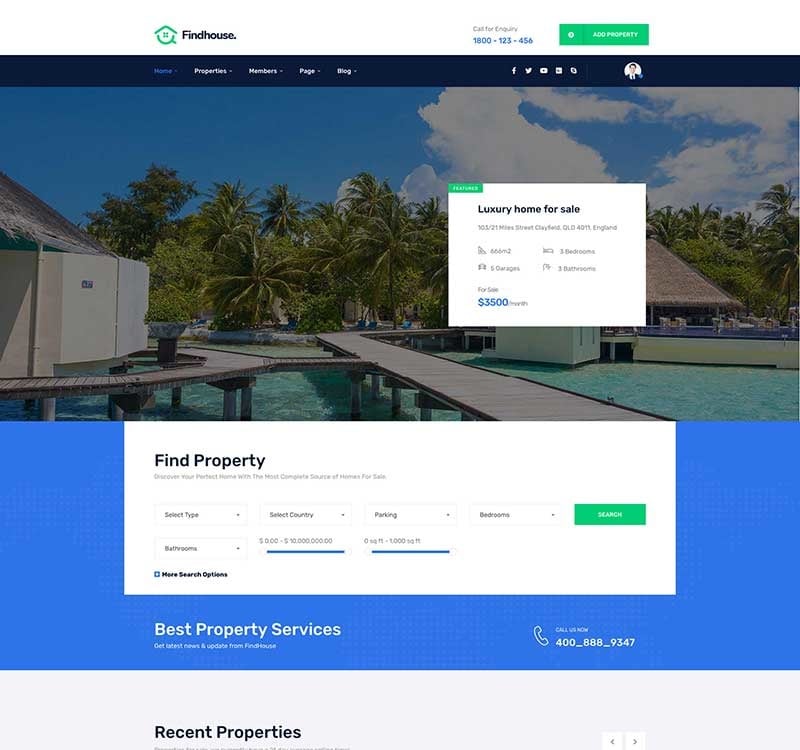Sure, here is a more detailed and cleaned-up version of the caption:

"A screenshot of the 'Find House' website, featuring a user-friendly interface. At the top, there's a 'Call for Inquiry' option with the phone number 800-800-1234. Below this, a green 'Add Property' button is prominently displayed. The navigation bar includes several drop-down menus labeled 'Home,' 'Properties,' 'Members,' 'Page,' and 'Blog.' Social media icons for Facebook, Twitter, and possibly YouTube are situated next to these. 

The main content of the screenshot features a high-resolution photograph of an opulent hotel room in a tropical setting, designed in a bungalow style. Beneath the image, a caption reads 'Luxury Home for Sale,' located at 'Something Street, Clayford, OLD 4011, England.' The listing details include 'Three Bedroom, Three Bathroom,' and the property is advertised 'For Sale at $3,500 per month.' Below this, a 'Find Property' link is visible. The image quality is somewhat low, making smaller text difficult to read, but it also advertises, 'Discover Your Perfect Home with the Most ... Source of Homes for Sale.'"